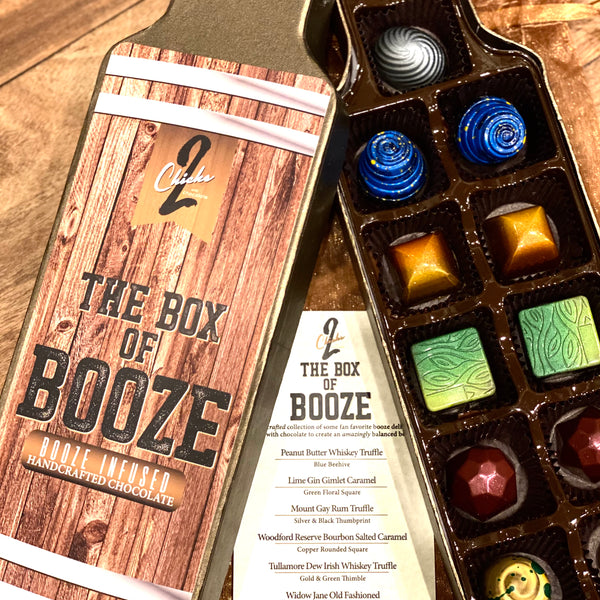This detailed photograph showcases a unique product called "Two Chicks, The Box of Booze," featuring booze-infused handcrafted chocolates. The box is designed in the shape of a liquor bottle with a lid that resembles a wooden barrel, complete with distinctive stripes representing barrel bands. The open box reveals an assortment of visually striking chocolates arranged in rows within brown plastic packaging. These chocolates come in various shapes such as squares, rounds, and a decahedron, and exhibit a palette of metallic colors including silver, gold, green, blue, and burgundy, some with intricate patterns like swirls and splatters. 

In the center, a paper insert provides detailed descriptions of each chocolate: blue beehive-shaped peanut butter whiskey truffles, green floral squares of lime gin gimlet caramel, silver and black thumbprint Mount Gay rum truffles, copper rounded squares of Woodford Reserve bourbon salted caramel, thimble-shaped Tullamore Dew Irish whiskey truffles in gold and green, and Widow Jane Old Fashioned truffles. The text on the insert, as well as on the packaging, emphasizes the artisanal nature of these indulgent treats, describing them as "booze infused handcrafted chocolates" that promise a sophisticated tasting experience.